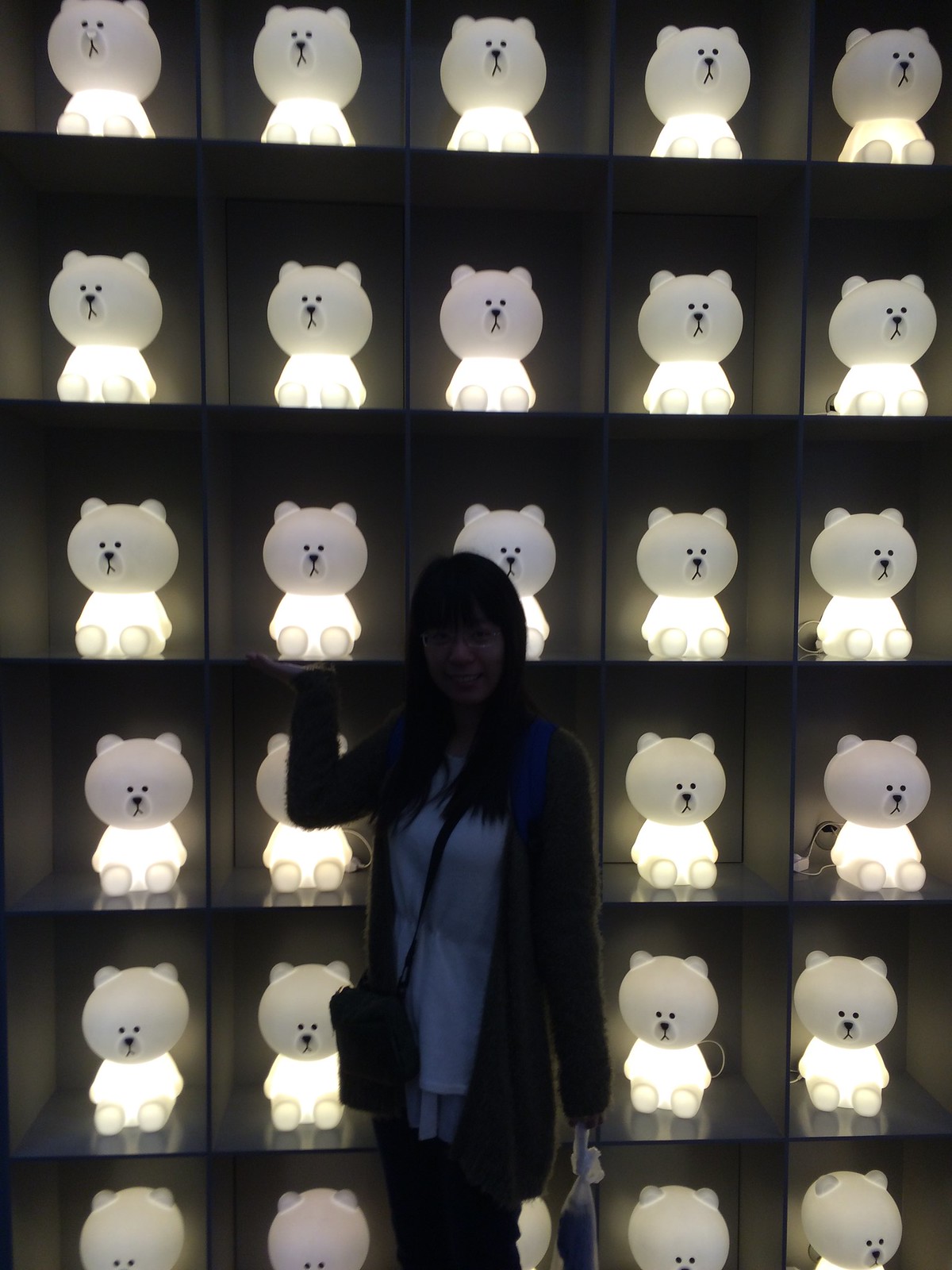The image depicts a wall-mounted shelving unit divided into individual compartments, each housing an illuminated teddy bear-shaped light figure. The shelving structure consists of six horizontal and five vertical sections, creating a total of 30 compartments, each separated by glass panels. Every teddy bear light, which emanates a soft, atmospheric glow, features black eyes and a snout detail, with most displaying black noses except for potentially one in the top left corner with a white nose. The bears sit with their feet stretched out in front of them, and each is connected to its own individual socket at the back.

Standing in front of this display is a Chinese woman with long dark hair, smiling at the camera. She is wearing glasses, a long gray sweater over a white blouse with a blue design, black pants, and a purse slung over her shoulder. In her left hand, she holds a white bag, while her right hand is extended upward as if presenting the illuminated teddy bears behind her. The combined elements create a serene yet lively atmosphere, with the glowing bears providing a notable ambiance to the scene.